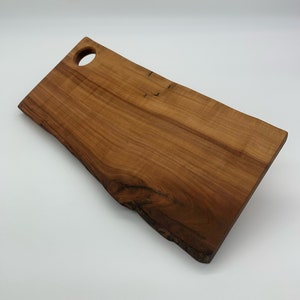This image features a slightly lopsided rectangular wooden cutting board with a hole in the top right corner, likely for ease of lifting or hanging. The board, resting against a plain white background, showcases a beautiful wood grain marked by different shades of brown and black. The wood transitions from lighter tones at the top to darker, almost burnt-looking marks at the bottom right, indicating possibly a knot or burnt edges. Distinctive lines enhance its texture, and the board appears thick and robust. While three edges are smooth, one edge retains raw, rustic imperfections, adding to its charm.